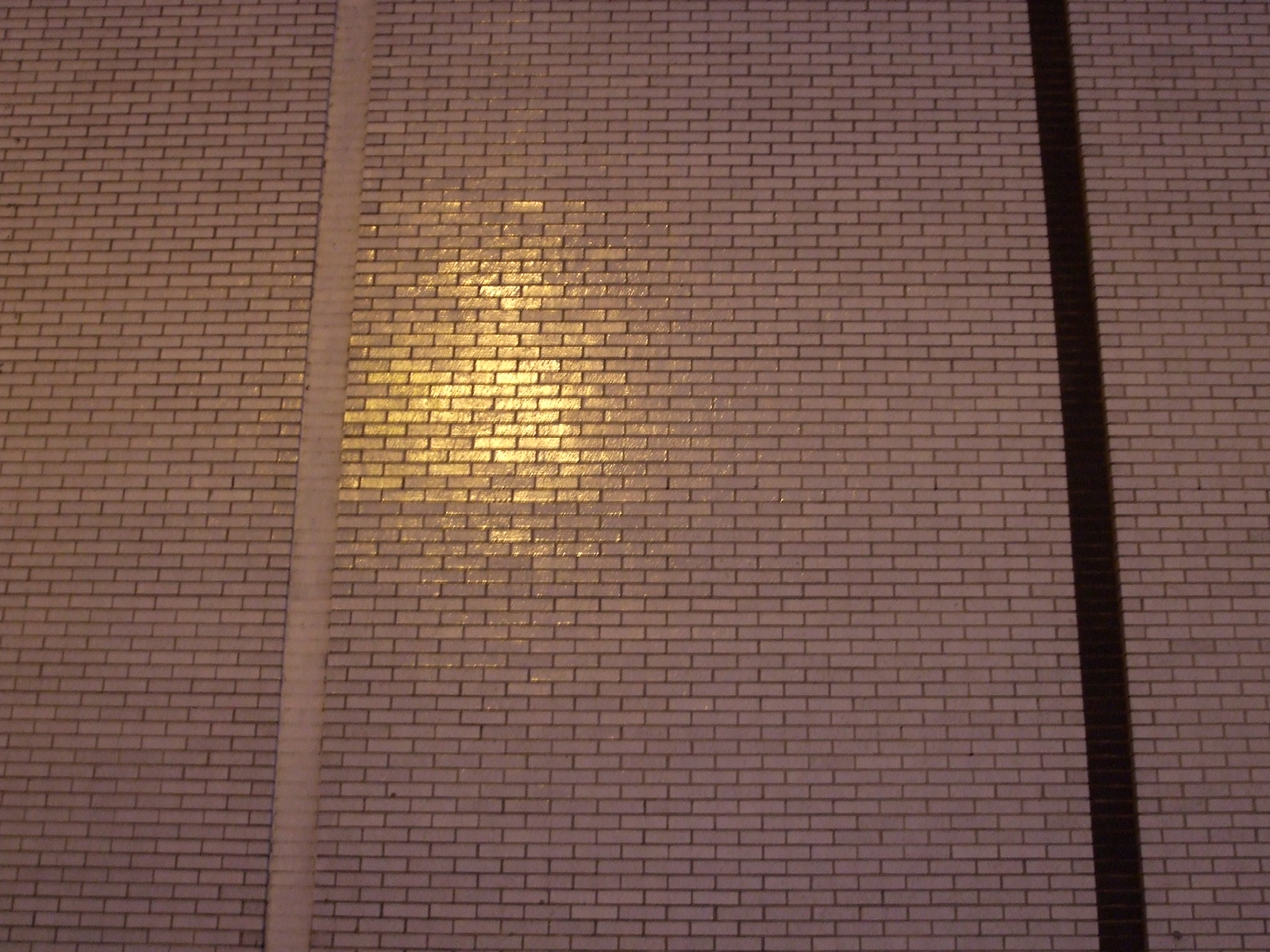This photograph captures a massive, glossy white brick wall that is part of a building. The wall is composed of thousands of small, white bricks, meticulously aligned with dark gray or black mortar between them. The wall is segmented by two distinct seams: a white seam on the left and a black vertical line on the right, which tilts slightly to the left. The bricks exhibit a shiny, reflective quality, suggesting they may be treated or polished. The wall is illuminated by a powerful, round light source—likely a street lamp—casting a yellow glow over a section of the wall near the white seam on the left side. This intense light accentuates the glossy texture of the bricks, creating a striking visual contrast against the dark separation lines, making the scene appear to be set at night.